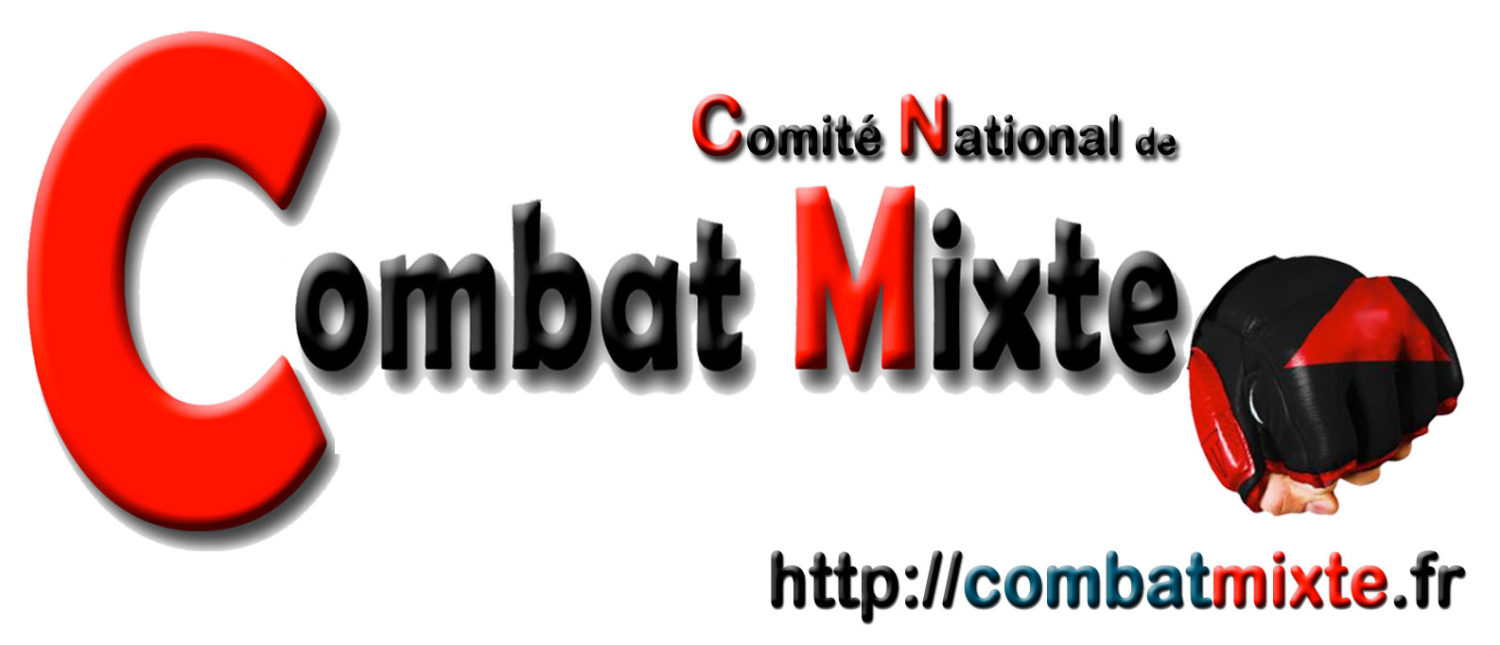The image features a dynamic logo designed for a website. Dominating the center is a large, bold red letter "C" followed by the word "combat" in black text. Adjacent to it, "mixte" is written with a moderately larger "M" in red, and the remaining letters in black. Above this central text, the phrase "Comité National DE" is displayed, where both the "C" in "Comité" and the "N" in "National" are highlighted in red, while the rest of the text is in black. To the right of "mixte," there is an icon depicting a fist wearing some sort of glove, adding a combative theme to the logo. The web address, "http://combatmxt.fr," is positioned in the bottom right corner and is color-coded for emphasis: "http" in black, "combat" in teal, "mixte" in red, and ".fr" back in black. The overall palette of the logo includes bold strokes of red, black, and teal, suggesting a strong and active presence, likely related to mixed martial arts.